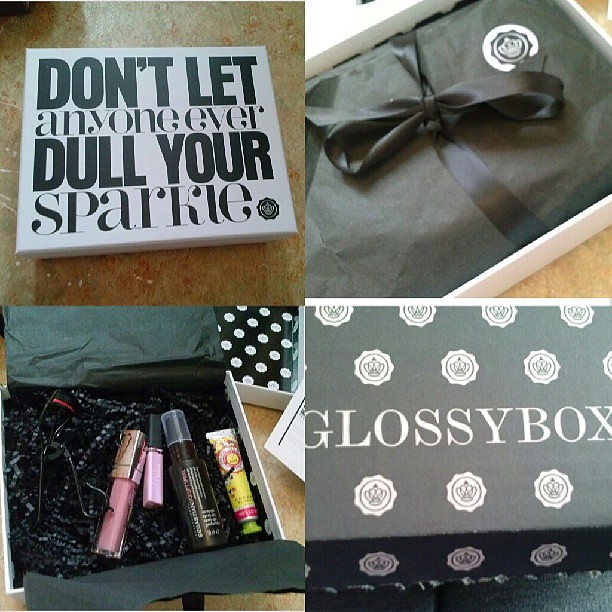The image is a detailed advertisement for the "Glossy Box" merchandise box. The top left corner features an inspirational sign reading, "Don't let anyone ever dull your sparkle." The box, prominently displayed in the other sections of the image, is black with a white and black crown emblem. In the top right, the box is shown with its lid removed, revealing black tissue paper and a neatly tied black ribbon. The bottom left section unveils the contents once the tissue paper is unwrapped: four cosmetic products, including glass and plastic tubes, nestled securely on soft, black packing material. The bottom right image showcases the box cover, emphasizing its elegant design with the crown logo and "Glossy Box" text.